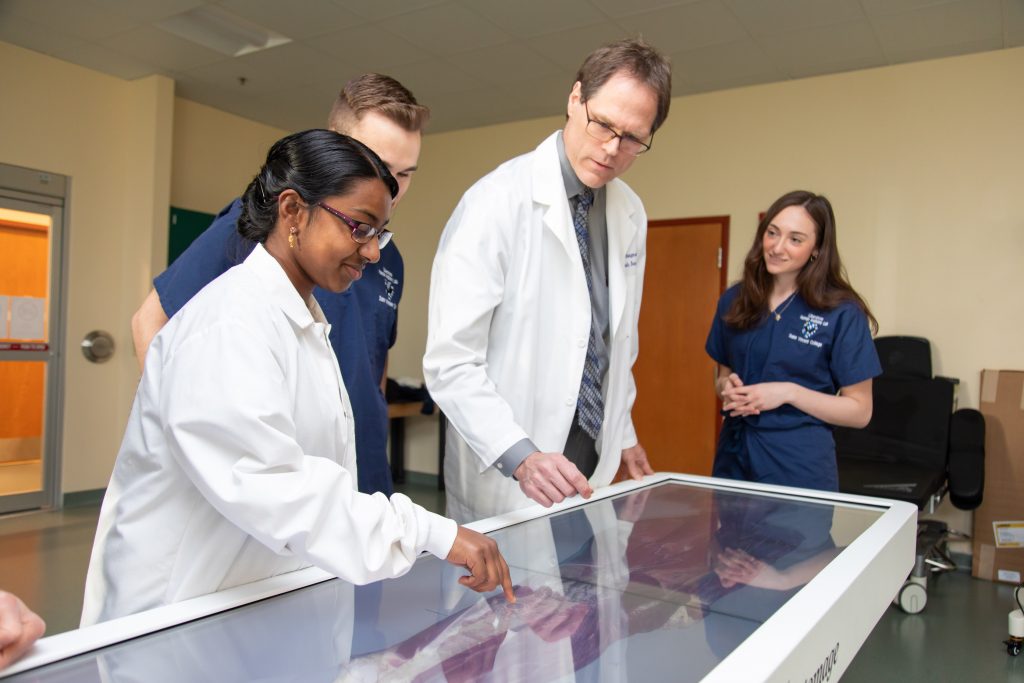The image depicts a group of medical professionals engrossed in examining something on or beneath a glass-covered desk. On the left, a Middle Eastern or Indian woman, dressed in a white lab coat, is smiling as she points at the glass surface, possibly a touch screen or a display case with a white frame. Behind her stands a tech worker dressed in blue scrubs, who also observes intently. Towards the right, another woman in blue scrubs smiles subtly, while a man in the center, wearing a gray shirt, tie, and a white lab coat, reviews the information being indicated. Both individuals in lab coats wear glasses, contrasting with the two in blue scrubs who do not. The background is a medical setting with cardboard boxes and some faint beige and brown accents, contributing a minimalistic appearance to the scene of scientific inquiry.